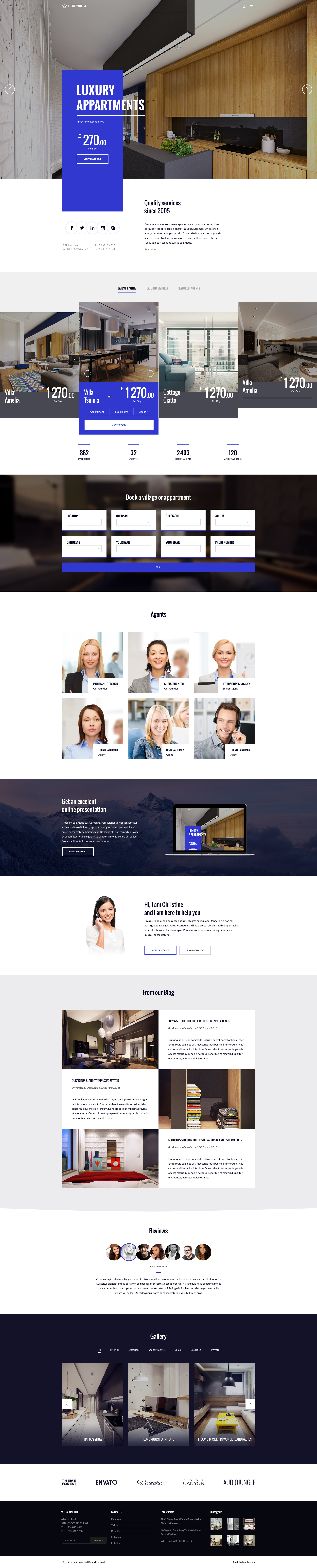The image depicts a slightly out-of-focus, stretched-out view of a full webpage. At the top, the header prominently displays the phrase "Luxury Apartments," alongside what appears to be an offer or price of "$270 each." Below this, there is a picture of a modern kitchen area, featuring brownish-stained cabinets in an open-plan layout. 

Following the header image, a section with a title and body text likely describes the apartments and amenities in detail. Beneath this descriptive text, there are four highlighted squares arranged in a row, each displaying different prices. The square that is in focus shows a price of "$1270" and seems to provide a glimpse into a potential living space, although the exact room type is difficult to discern.

Further down, there are eight long rectangles, each containing text, and a single, lengthy, narrow rectangle that spans the width of these eight. The content of these rectangles is unclear due to the image quality.

Towards the bottom of the page, there are six headshots, mostly of women with one male, presumably the team or residents. Adjacent to these headshots, another section features a woman holding her ear in one picture and multiple spaces with three descriptions in another.

Overall, the webpage offers a detailed presentation of luxury apartments, featuring kitchen imagery, pricing options, and possibly testimonials or team member introductions.